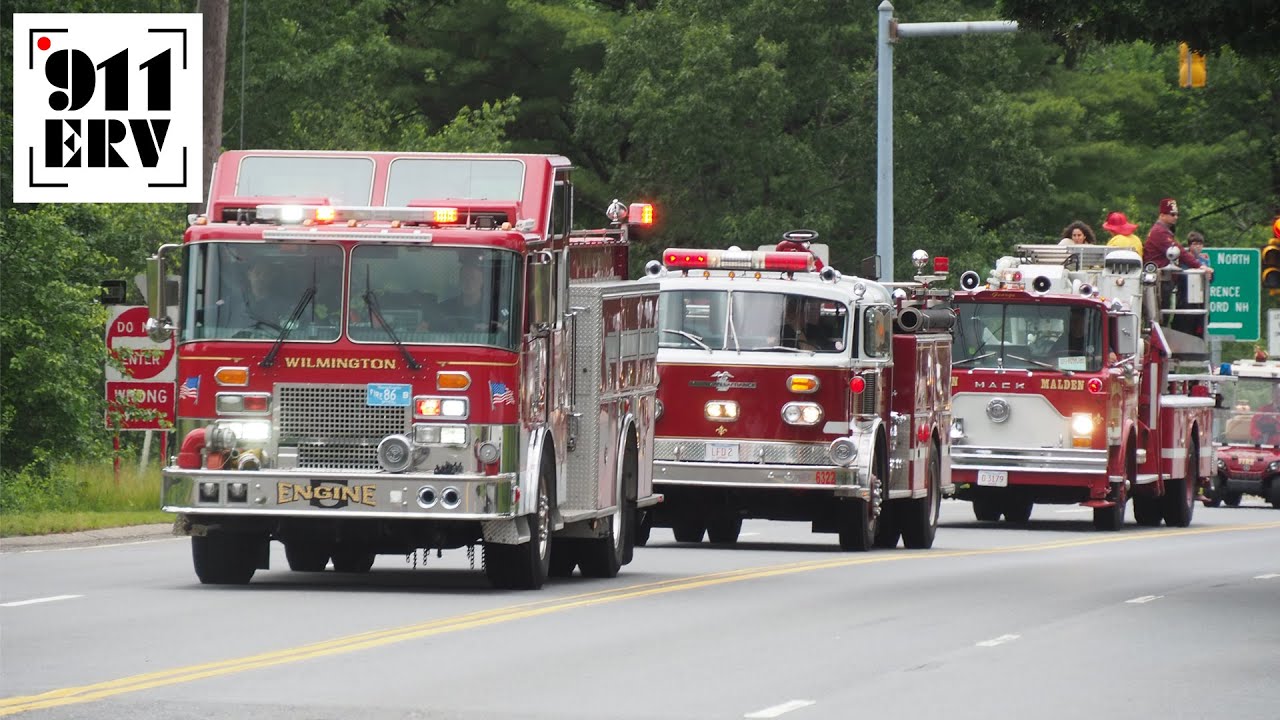This daytime photograph depicts a procession of three fire trucks driving closely together down a four-lane road, delineated by a yellow double line, with dense, dark green foliage forming the backdrop. The trucks, all in red and white, are moving from the left towards the right of the image. The first truck prominently displays the words "Wilmington" and "Engine" on its front. The third truck features multiple individuals atop it, including a person in a red fire hat and yellow jacket, a woman with dark black hair, and a man in a dark jacket. The fire truck lights are illuminated, suggesting a parade or tour-like event rather than an emergency response. A logo reading "911 ERV" with a red dot and black frames around each corner is visible in the upper left corner of the rectangular photograph.